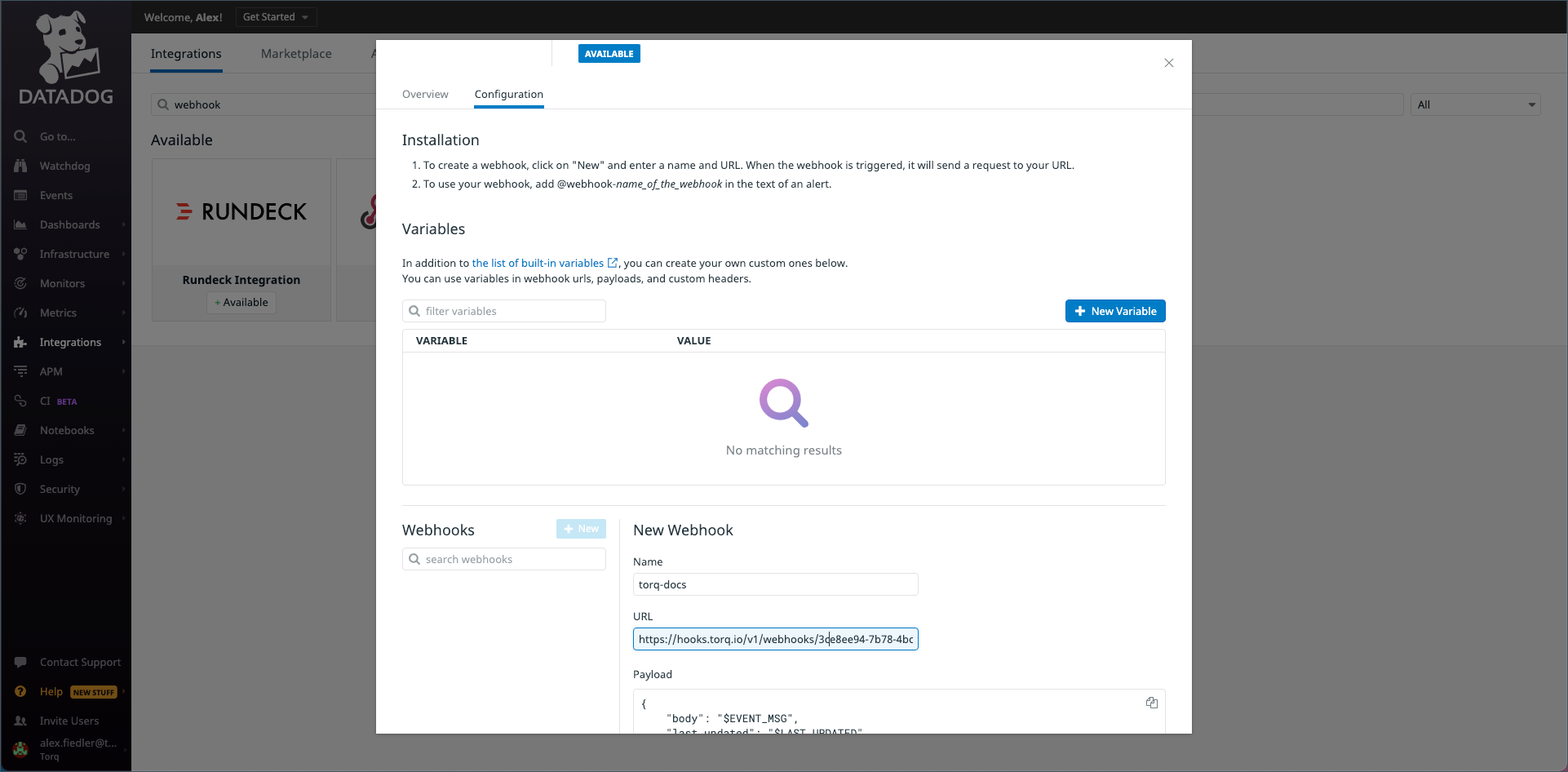The image depicts a computer interface with a screenshot as the main focus. In the background, a computer screen is visible with a black area on the left side. At the top left corner, there's an image of a dog holding a picture in its mouth, labeled "data dog." 

A vertical list of options is present on the left, partially visible. In the central part of the screenshot, there are sections titled "Integrations" and "Run Deck" to the right. A white pop-up window dominates the middle of the screen, featuring a blue banner at the top that says "Available." 

Within this pop-up, there are two main headings: "Overview" and "Configuration," with "Configuration" underlined. The text within the pop-up provides instructions for creating a webhook. It reads: "To create a webhook, click on 'New' and enter a name and URL. When the webhook is triggered, it will send a request to your URL. To use your webhook, add the webhook name to the text of an alert." 

Further down in the pop-up, another section titled "Variables" explains that, in addition to built-in variables, users can create custom ones. It mentions that these variables can be used in webhook URLs, payloads, and custom headings.

A box labeled "Variable" and "Value" with a search icon displays "No matching results." Underneath this, there's a section labeled "Webhooks" with a heading "New Webhook" next to fields for "Name" and "URL."